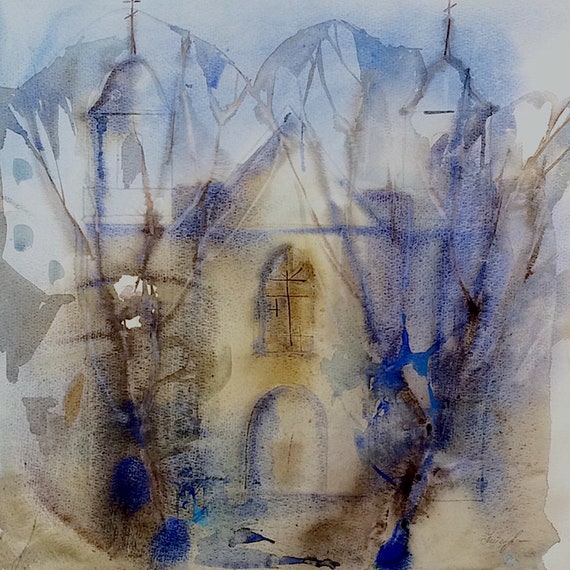This artwork is a subdued, somber painting or collage dominated by muted blues and browns. Central to the piece is the vague, dreamlike outline of a building that resembles a church or a mission, characterized by its A-frame roof, a curved door, and an arched window above it, possibly boarded with horizontal lines. Flanking the main structure are ambiguous forms, including towers topped with steeples and crosses, hinting at a religious significance. Behind the building, a hazy, light blue sky with rugged mountain silhouettes extends, adding to the ethereal atmosphere.

Emanating from the church are abstract splotches and patches of royal blue and gray, creating a sense of obscurity and fluidity. These blotches might suggest the presence of trees or other forms but remain indistinct and out of focus, enhancing the painting’s mysterious and somber character. Superimposed over this background, there appear to be hanging garments—suits, jackets, a dress, and a slip—that drape and overlap, contributing to the sense of layering and depth.

Overall, the artwork evokes a feeling of uncertainty through its muted palette, blurred details, and juxtaposition of religious architecture with everyday objects, all set against a soft, blurred background.